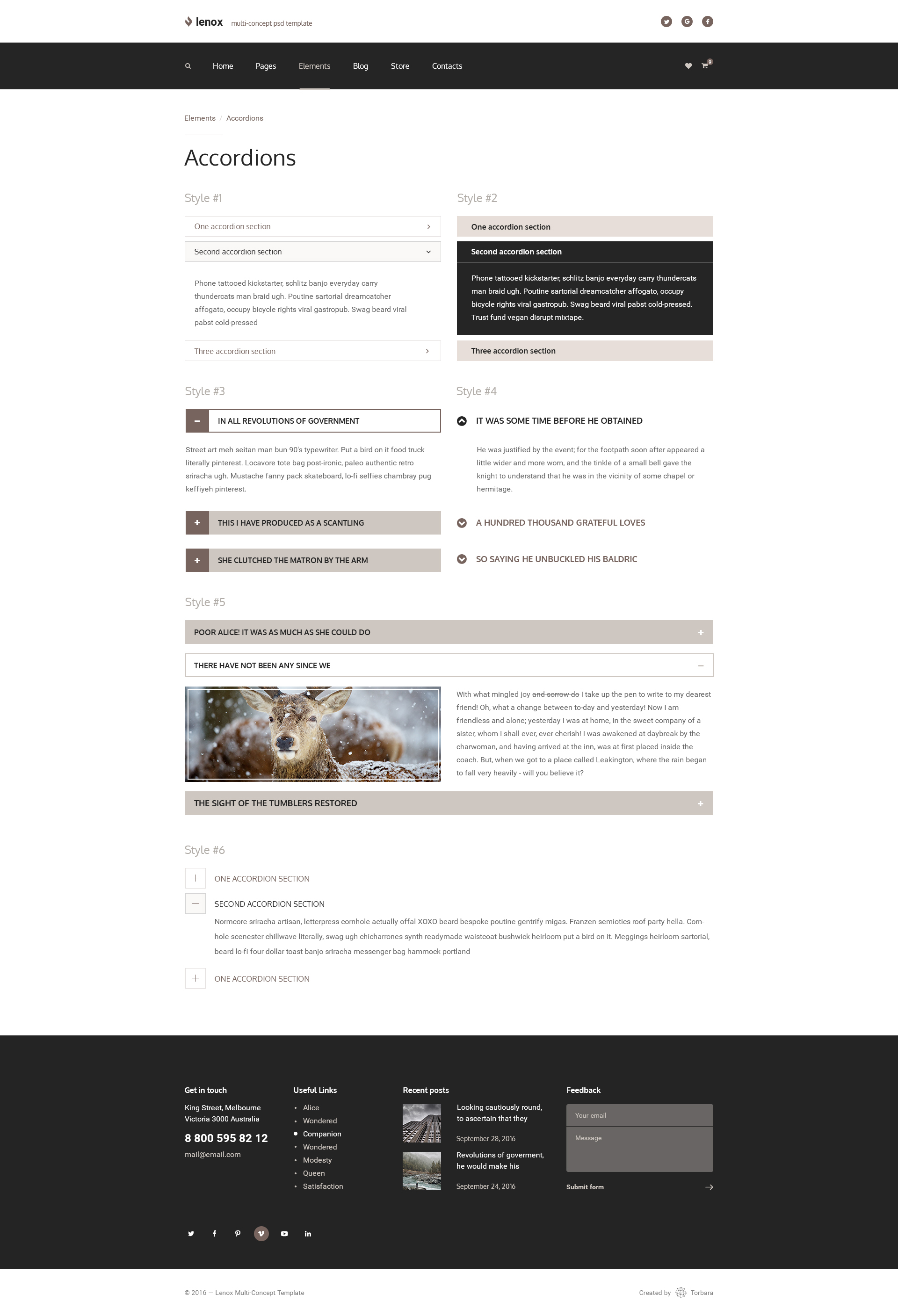The image prominently displays a website layout with "Linux" written in black at the top left corner. Below this header, a navigation bar with a black background lists several categories: Home, Pages, Elements, Blog, Store, and Contacts. The "Elements" category is currently selected, indicated by a white horizontal line beneath the word. To the left of "Home" is a magnifying glass icon, and to the right of the categories are heart and shopping cart icons.

Centered at the top left of the main content area, the image reads "Elements" followed by "Accordions" in a slightly smaller font. Above these words, in larger text, it repeats "Accordions." Below, there are different accordion styles labeled as Style 1, Style 2, Style 3, and Style 4, each enclosed in a square-like box and featuring descriptive text about their respective styles.

In the middle bottom portion of the image, Style 5 is showcased. It includes a picture of a deer with accompanying text to the right. This text reads, "There have not been any since we," followed by "Poor Alice, it was as much as she can do." Beneath the deer image, the text "The sight of the tumbler is restored" is visible.

Finally, at the very bottom of the image, Style 6 is presented with two sections labeled as "one accordion section" and "second accordion section."